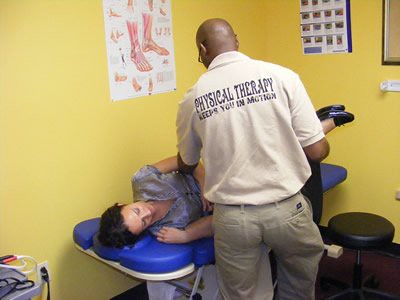The image depicts a scene inside a medical clinic with bright yellow walls adorned with various anatomical diagrams, including one of feet and ankles. In the center, an African American man, identifiable as a physical therapist, wears a beige polo shirt with the phrase "Physical therapy keeps you in motion" on the back, along with khaki pants. The therapist is standing with his back to the camera, possibly adjusting or examining the limbs of a woman lying on her side on a blue, spongy examination table. The woman has dark hair, a blue short-sleeved blouse, and black shoes without visible socks. To the therapist's left, some equipment is plugged into the wall on a table, and a black circular stool sits in the lower right corner of the image. A small mirror can be seen in the upper right corner, adding to the clinical setting.